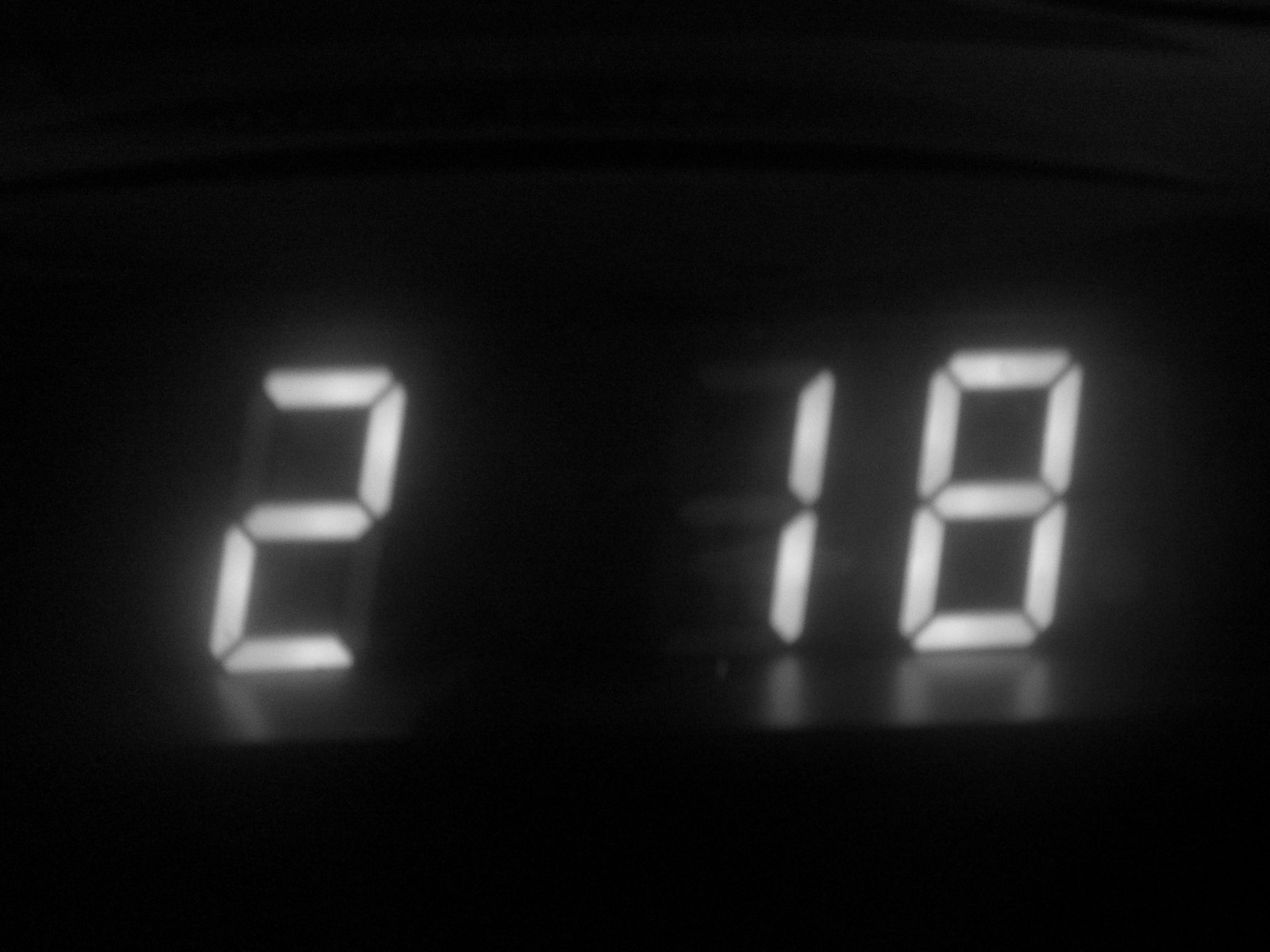A close-up image captures an electronic clock display against a completely black background, likely taken at night. The focus is on the illuminated digital numbers "2:18" which stand out starkly in bright white. The display appears to be situated on a small ledge, with the light from the digits casting a subtle reflection on its surface, revealing faint outlines of the numbers. Additional faint lines emanate from the lit digits, adding a soft glow around the display. The surrounding darkness emphasizes the illuminated numbers, creating a stark contrast and drawing attention solely to the time display.